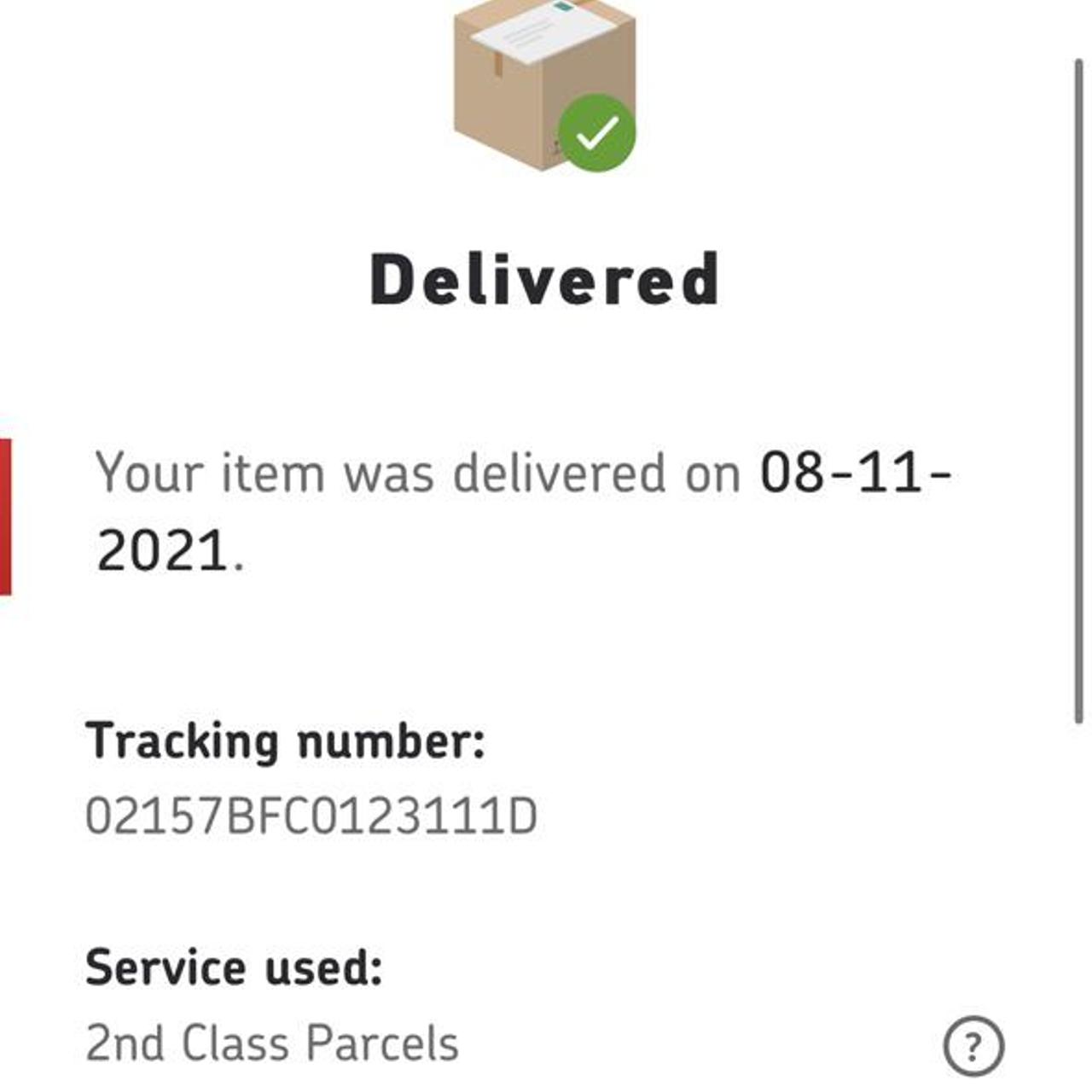The image displays a delivery confirmation dialogue. At the top center, there is a three-dimensional icon of a parcel box with a label on it. Adjacent to this box is a circle featuring a white checkmark, indicating that the item has been delivered. Directly below, in large black font, the word "Delivered" is prominently displayed.

Beneath this, on the left-hand side, there is a red vertical line. To the right of this line, text in black and gray states: "Your item was delivered on 08-11-2021", with the date in black and the rest of the text in gray. Following this, a black heading reads "Tracking Number", followed by the tracking code "02157BFC0123111D" in gray text.

Next, under another black heading labeled "Service Used", the service is specified in gray as "Second Class Parcels". To the right of these details, there is a small gray circle containing a question mark for additional help. A scroll bar is visible along the right side of the image.